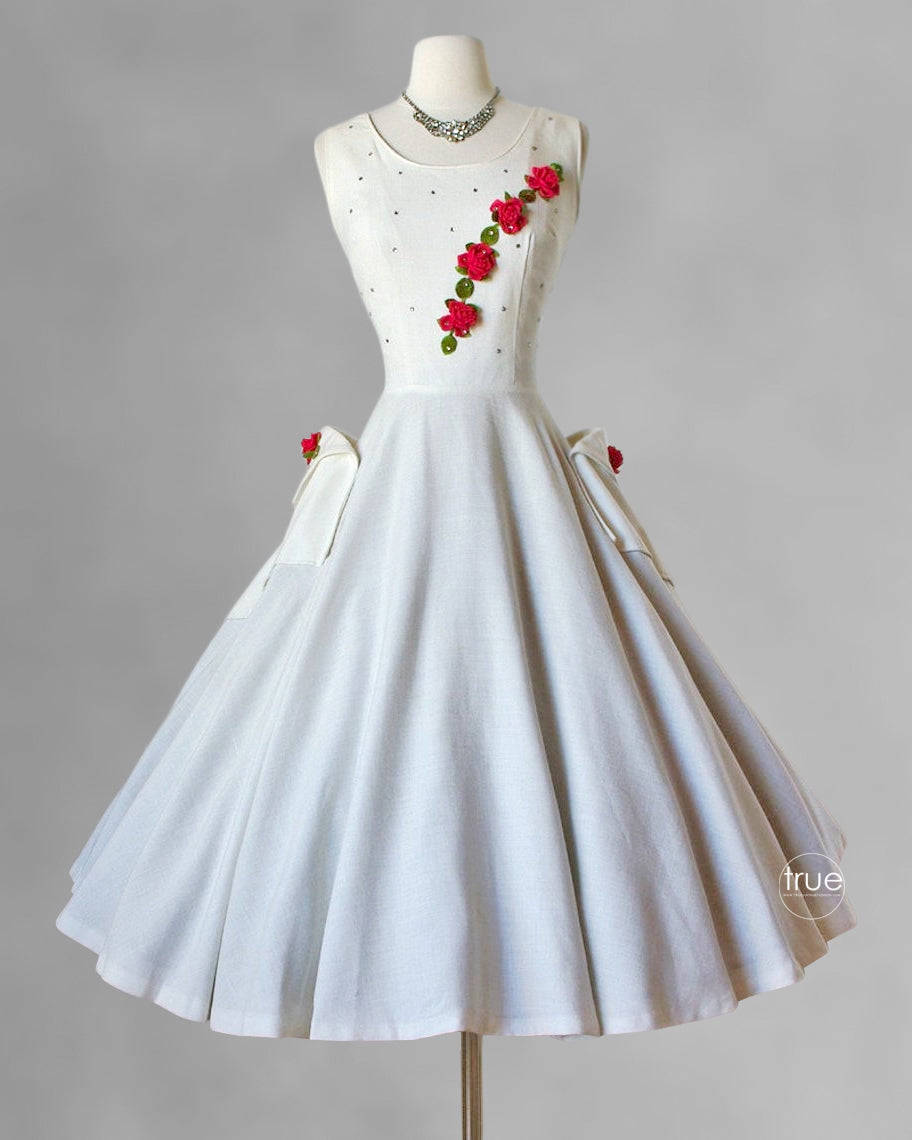The image showcases a detailed photograph in full color, oriented vertically, set against a plain gray background. The focal point is a white, sleeveless dress displayed on a mannequin, designed for a party or spring affair. The dress features a fitted bodice decorated with small black polka dots and adorned with a line of four red fabric roses extending diagonally towards the right side. The voluminous, frilly skirt flares out dramatically, emphasizing two large white pockets, each embellished with a small red fabric rose. Adding to the ensemble, the mannequin is accessorized with a striking silver necklace, potentially embedded with crystals or diamonds, enhancing the overall decorative and elegant appearance of the outfit.